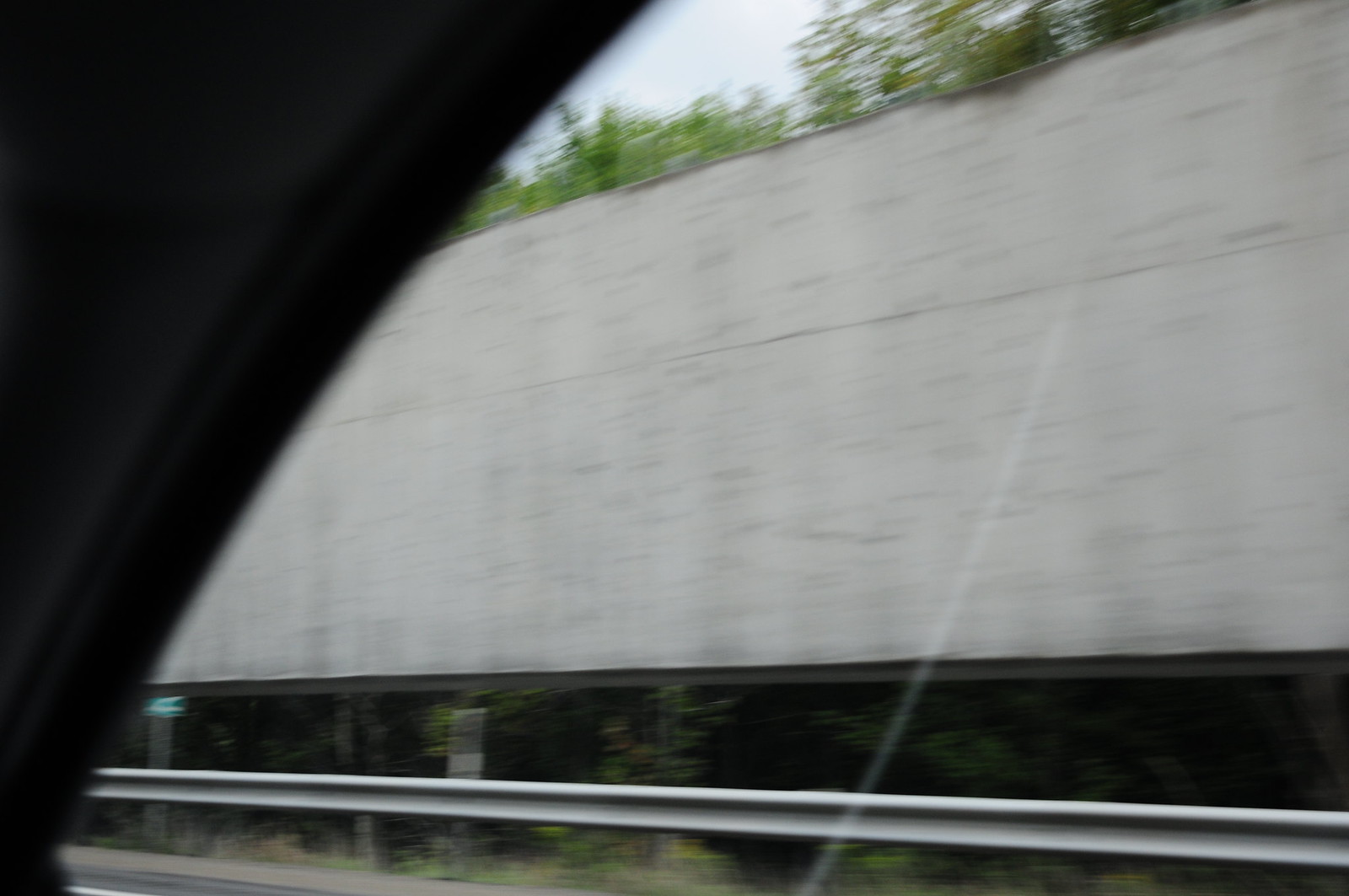This photo, captured from a moving vehicle, shows a dynamic scene with a metallic guardrail on the right side of the frame. Just beyond the guardrail, there is a white rectangular structure, its exact purpose uncertain—possibly a wall or maybe an old sign—accented with faint black streaks. The motion blur from the moving car renders the structure indistinct. In the background, lush dark green trees rise up, adding depth to the scene. Above, a portion of the sky peeks through, providing contrast with the greenery. Additionally, a small part of the car's interior is visible in the shot, hinting at the perspective from which the photo was taken.